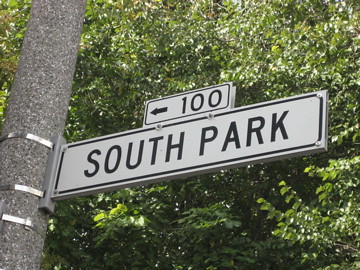The image features a background dominated by lush green trees, indicating a daytime setting with sunlight illuminating the foliage. Prominently positioned on the left side is a cylindrical pole, appearing thick and primarily gray with white specks and some black markings. The pole is truncated at the top and bottom edges of the image, leaving its full length indeterminate. This pole is encircled by three silver bands that support two distinct rectangular signs. The larger sign, which is white with a black border, displays "SOUTH PARK" in bold, uppercase black letters, extending horizontally. Positioned above it is a smaller, similarly designed white rectangle bordered in black, containing a black arrow pointing to the left and the number "100" in bold black text. The detailed contrasts among the pole, its mountings, and the signage, coupled with the verdant background, create a vivid, structured composition.